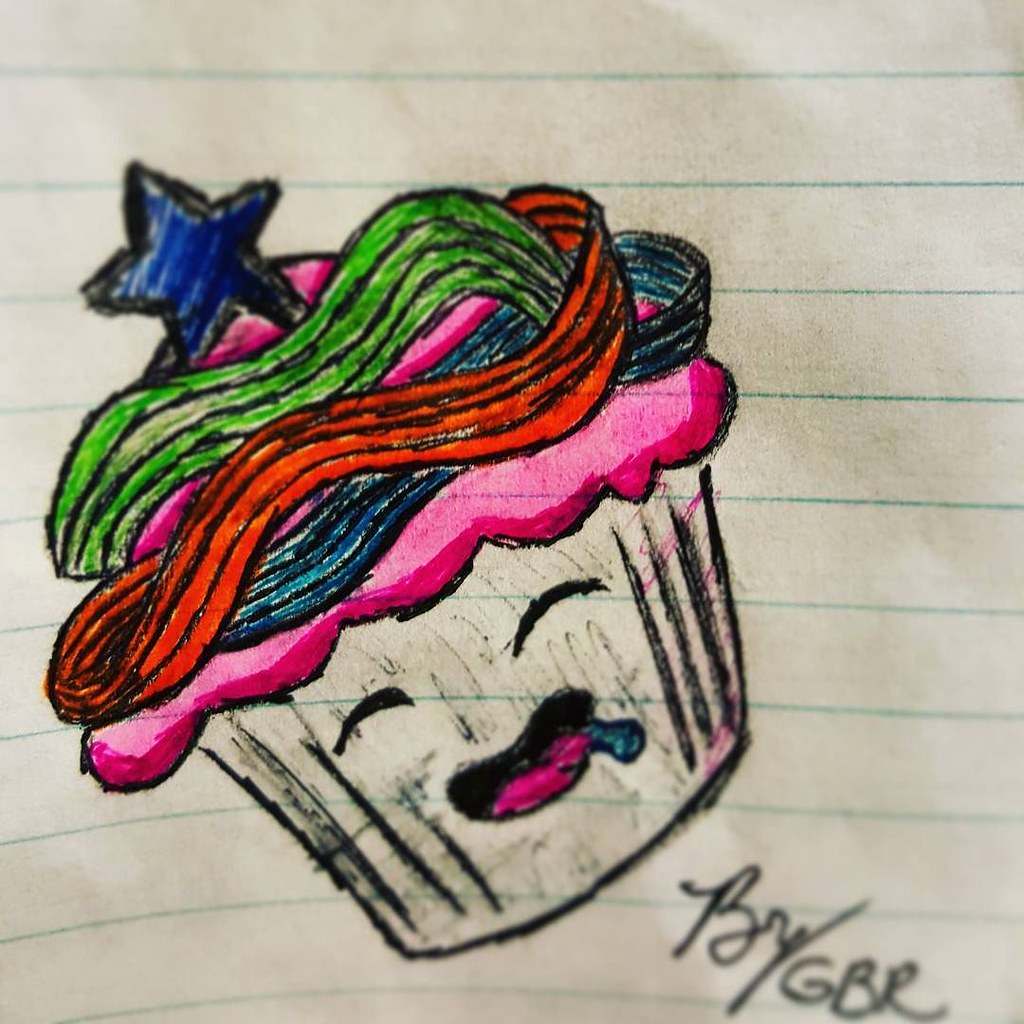The image depicts a detailed close-up of a whimsical sketch on a white, lined piece of paper. The paper features blue horizontal lines and dark smudges from the drawing process. In the bottom right corner, there is a distinctive signature in black ink, reading "BR / GBR" in capital letters. 

The centerpiece of the sketch is a charming cupcake with anthropomorphic features on its liner. The liner is crisply drawn with white vertical streaks, resembling the folds of a cupcake wrapper. The cupcake sports a cheerful face: its eyes are depicted as black, curved arches giving it a lively expression, while its open mouth reveals a pink tongue and a droplet of blue drool, adding a playful touch.

The top of the cupcake is decorated with layers of vibrant icing. The base layer is pink, adorned with ribbons of dark blue, orange, and green icing, creating a colorful contrast. At the summit of the icing sits a small dark blue star, completing the enchanting design. The medium used for the drawing appears to be a mix of crayon and black pencil, lending it a textured and vivid appearance.